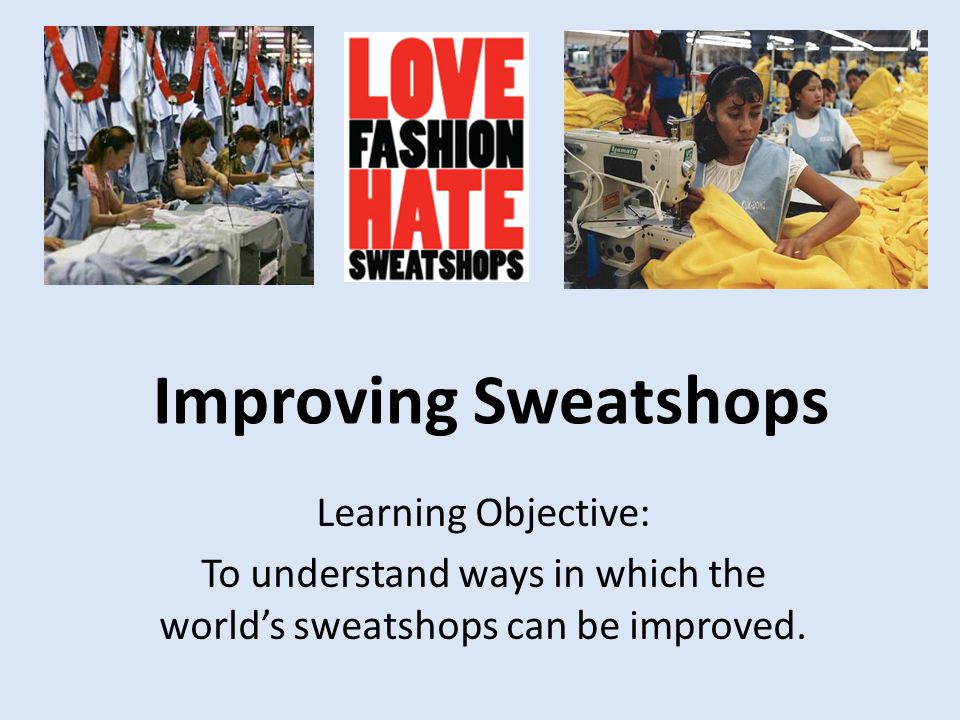The image is a presentation slide with a light blue background. At the top, there are two photographs: the left one depicts a group of women seated at tables, surrounded by various garments and materials, deeply engaged in sewing activities. Clothes are visibly scattered on their tables and hanging behind them. The top right photograph shows another group of women, some in blue and white uniforms, operating sewing machines to produce garments. 

Between these two images, there is a rectangular section with a white background displaying bold text in alternating red and black colors. The text reads, "Love Fashion Hate Sweatshops." Below these photographs and the text, at the bottom of the image, are the words "Improving Sweatshops" followed by "Learning Objective: To understand ways in which the world's sweatshops can be improved." The overall presentation setup and the arrangement of these elements, along with the varied colors including white, red, black, brown, pink, green, orange, yellow, and light blue, suggest that this is part of a PowerPoint presentation aimed at educating about improving working conditions in sweatshops.